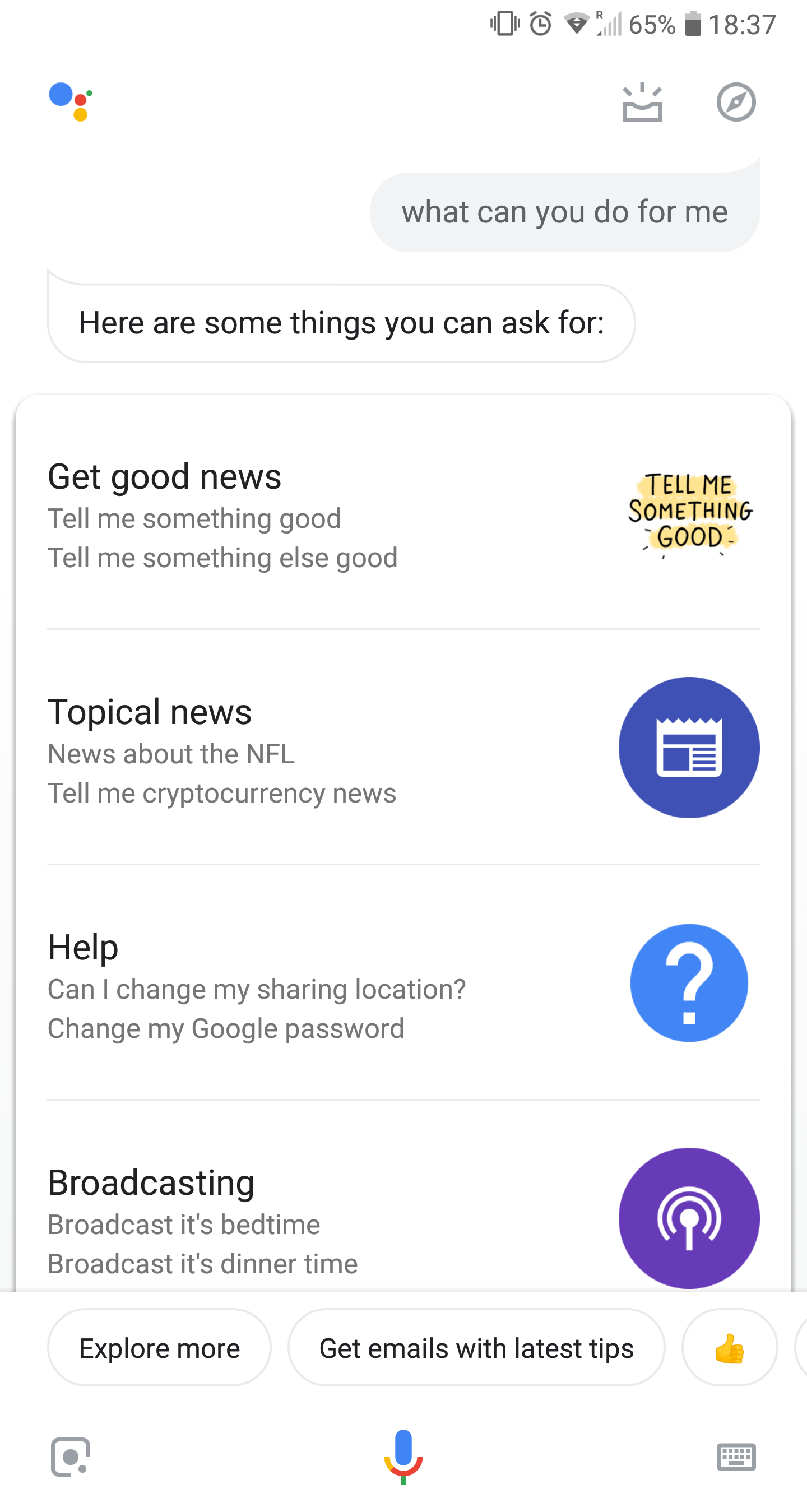This is a screenshot of a smartphone interface with a predominantly white background. In the bottom-left corner, there’s a blue circle, and further down to the right, there is a smaller red circle. Below the red circle, there is an even smaller yellow circle. Moving to the top of the screen, in the right corner, there is black text displaying "18:37" alongside a battery icon indicating 65% charge, one bar of internet signal, and a Wi-Fi connection icon. There are also alarm and vibrate icons.

Towards the bottom right section of the interface, there is a white circle with a gray border containing a line ascending from left to right. Above this, there is a small rectangle with three lines above it, each pointing in varying directions: up, upright, and up-left. Below is a gray speech tab containing the text "What can you do for me" in black. To the left, there is another white speech tab with a gray border that reads "Here are some things you can ask for" in black font.

Further down, on the left side, bold text reads "Get Good News," with two lines of regular-sized text beneath it. On the right, bold black text says "Tell me something good" with a tan overlay. Below this, the left side displays "Topical News" in a bold font, followed by two lines of information. On the right side, there is a dark blue circle with a paper icon inside it.

On the left side again, bold text reads "Help," with two lines of text underneath. On the right side, a light blue circle contains a question mark. Further down, left-aligned bold text says "Broadcasting," with two lines of text underneath, while on the right, a purple icon with a white line and two sideways, upside-down "C" shapes is visible.

In the center of the interface, there is a blue voice icon. To its left is a black camera icon, and to its right is a black calendar icon. Underneath these, several white tabs display various functions: "Explore More," "Keep emails with latest trip," and a tab with a thumbs-up icon.